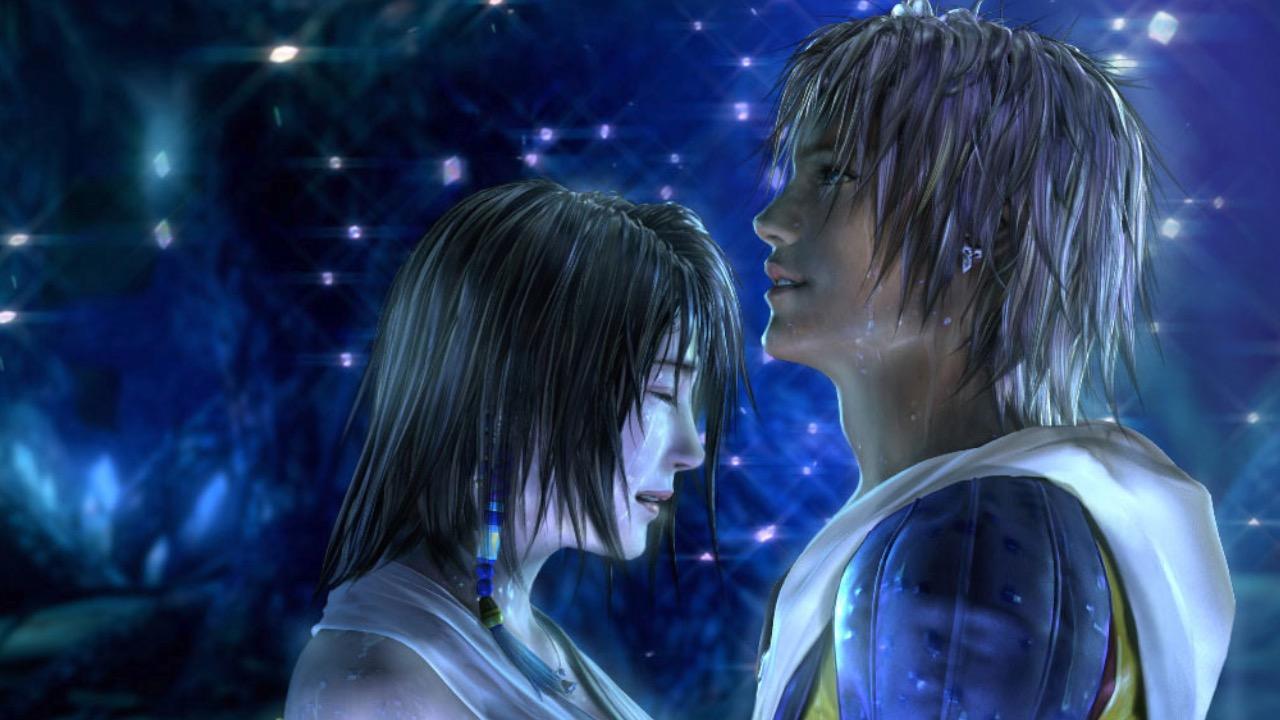The image depicts a poignant and intimate moment between two highly realistic animated characters, reminiscent of the modern Final Fantasy games, specifically Final Fantasy X. The female character, positioned in the foreground on the left side of the image, has straight, slightly wet hair and wears a sleeveless white top. She appears teary-eyed, with a long beaded earring adding to her delicate appearance. The male character, standing on the right, has wet hair as well and dons a multi-colored outfit consisting of blue, red, yellow, and white, with a poofy, cape-like feature on the shoulders. He also wears a smaller earring. His contemplative expression, as he looks away from the female, contrasts with her direct gaze. They are closely embracing, with the female's head reaching up to his nose. The background is a dreamlike blue filled with sparkling white lights and crystalline water droplets that shimmer, creating an ethereal atmosphere. The hues of blue, yellow, white, beige, tan, black, and gray blend harmoniously to enhance the emotional depth of the scene.